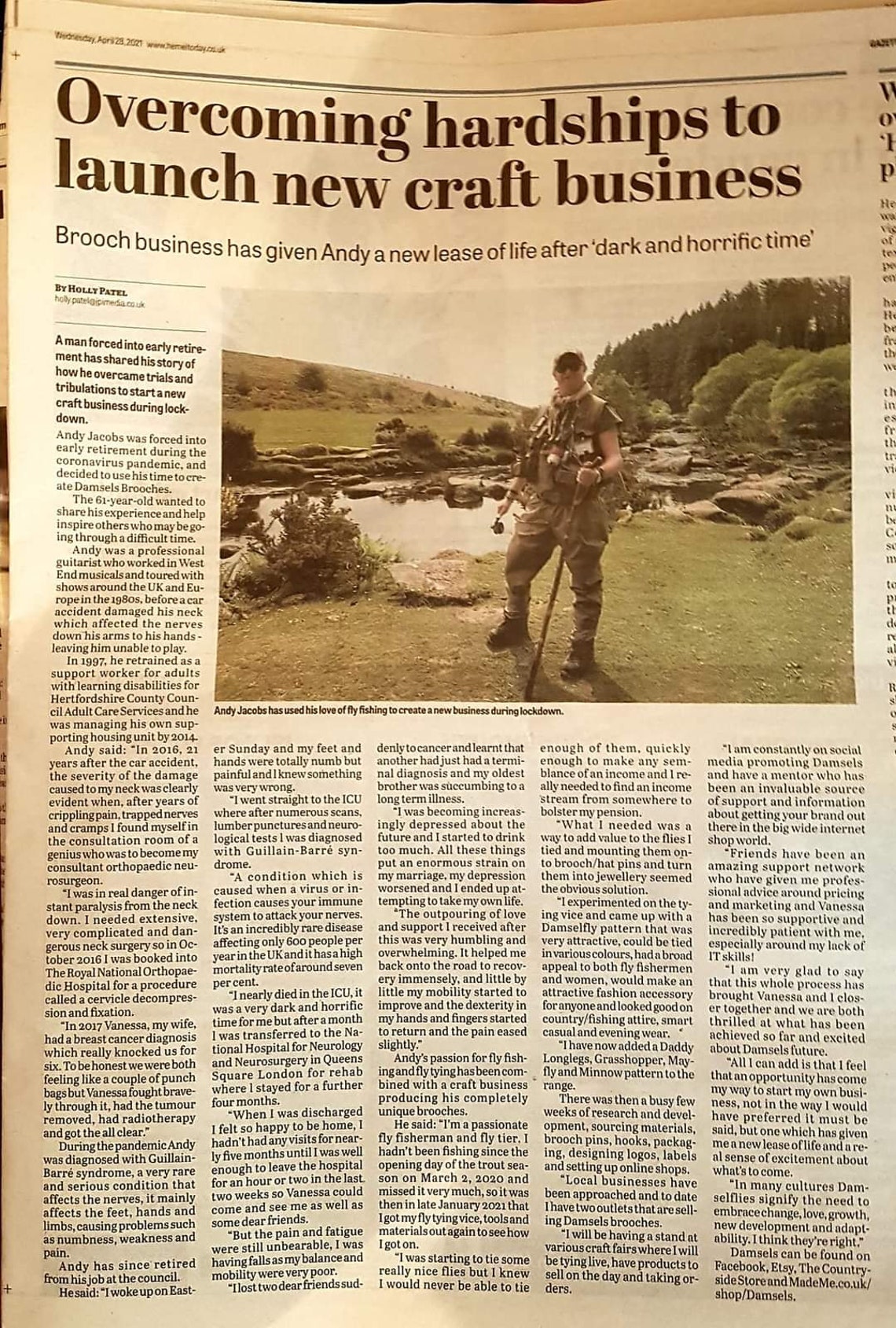This is a detailed photograph of a physical newspaper page displayed on a website. The image vividly captures the tactile imperfections of printed media: visible crinkles, areas where ink has smeared over a color photograph, and the subtle browning that suggests aging paper. The page has a slight fold at the top, indicating it has been handled. Registration marks, including a small plus sign in the upper left corner, are noticeable, along with two green bars at the top of the page.

The headline reads, "Overcoming Hardships to Launch New Craft Businesses." Featured prominently beneath the headline is an image of a man equipped for the outdoors. He's wearing hiking gear, including boots, a hiking pole (or possibly a fishing pole), sunglasses, and various items strapped around his chest and neck. He stands in a grassy area beside a stream, with a forest and hills forming a picturesque backdrop.

The article, penned by Holly Patel, begins with bold text: "A man forced into early retirement has shared his story of how he overcame trials and tribulations to start a new craft business during lockdown." It is composed of five tightly packed columns. The caption beneath the photo identifies the individual as Andy Jacobs, noting that he has leveraged his passion for fly fishing to establish a new business during lockdown. There is some ambiguity about whether the pole he holds is for hiking or fly fishing, but it is clear from the joyful expression on his face that he is thoroughly enjoying his endeavors.